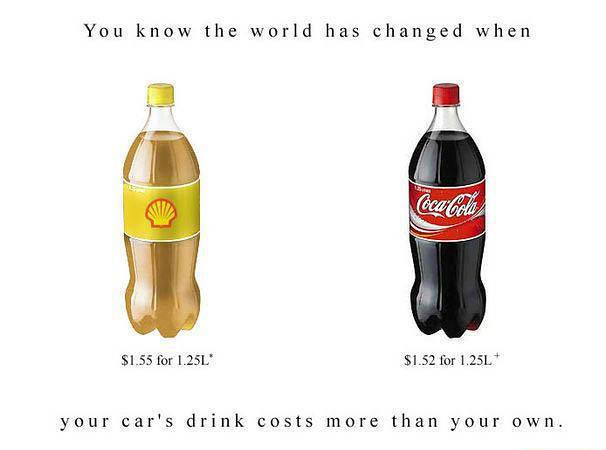This meme image is set against a white background and features black text at the top, reading, "You know the world has changed when," and at the bottom, "your car's drink costs more than your own." At the center, two plastic bottles stand side by side. On the left is a 1.25-liter bottle with a gold liquid inside, a yellow cap, and a yellowish-gold label adorned with the Shell gasoline logo—a yellow shell with a red outline. Below this bottle, it says "$1.55 for 1.25 liters." To the right is a 1.25-liter Coca-Cola bottle filled with a dark liquid, featuring a red cap and the iconic red label with white "Coca-Cola" text in swirling, underlined font. Beneath this bottle, it says "$1.52 for 1.25 liters," with a small star indicating a potential footnote, though no additional information is provided.